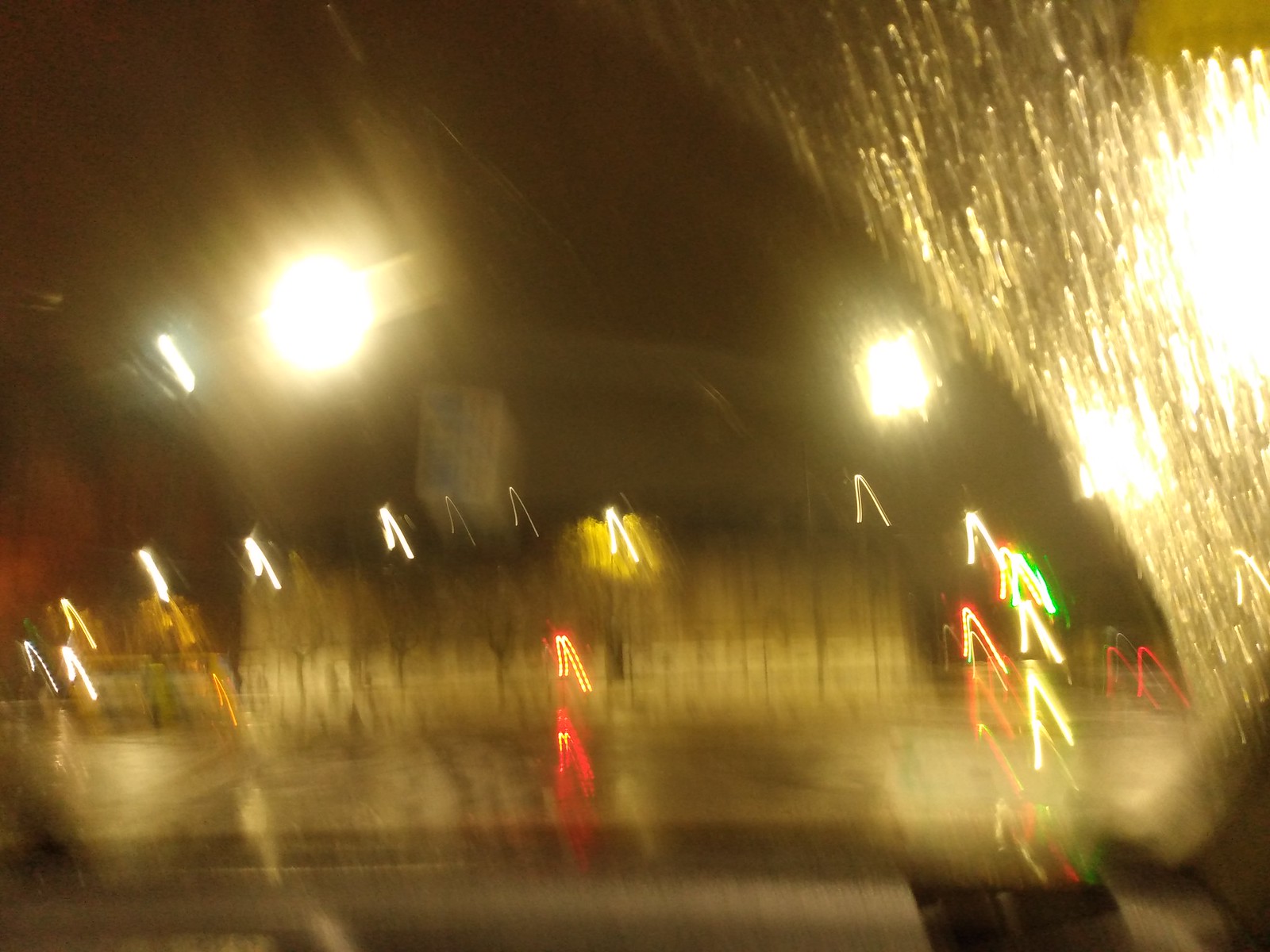A photograph taken through a car's windshield on a rainy night captures a blurred and out-of-focus scene. The image displays the car's dashboard at the bottom, characterized by a light gray bar stretching horizontally. Distinctly, the arc formed by the windshield wiper is visible, sweeping a semi-clear path through the otherwise rain-streaked glass. In the upper right corner, streaks from raindrops create a scattered pattern. Beyond the windshield, a wet, dimly lit street is barely discernible. Two large, bright white circles, possibly streetlights, dominate the background, while numerous small, upside-down V-shaped lights—in white, green, and red—suggest reflections and movements, adding to the chaotic, almost dreamlike atmosphere.